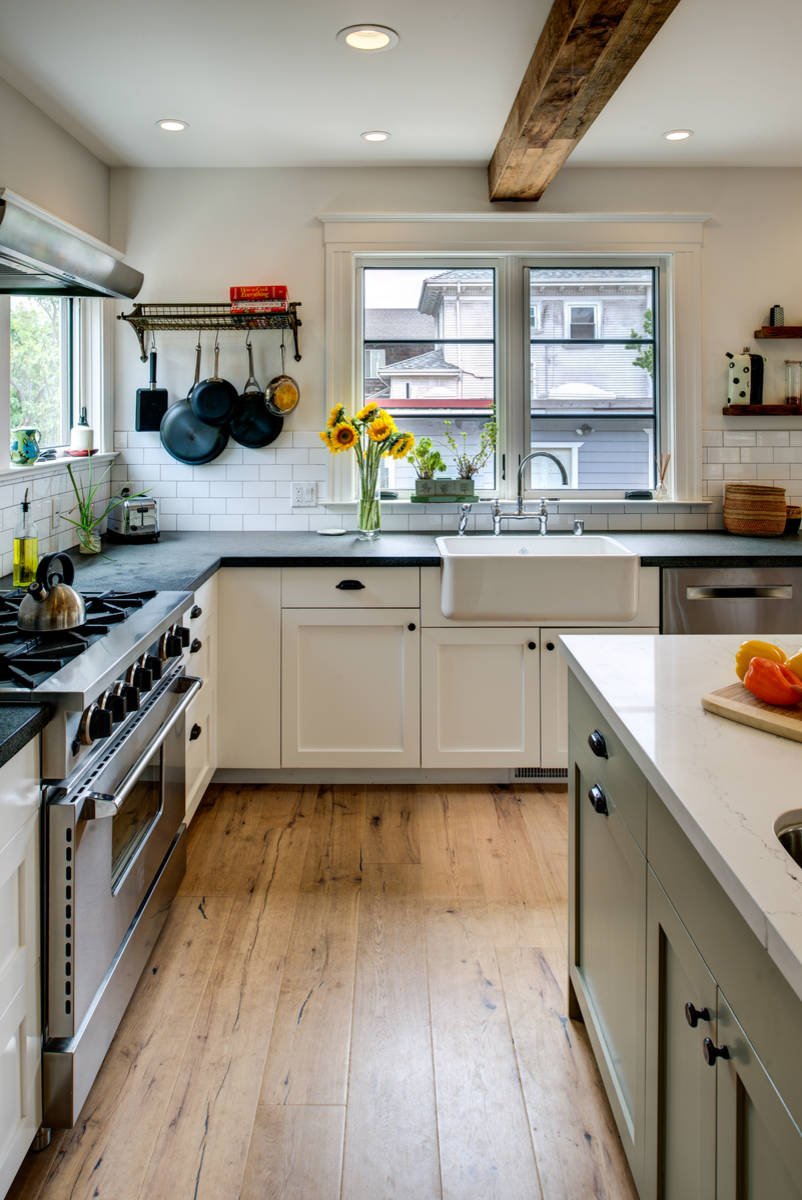The kitchen exudes a charming country home vibe with its light hardwood plank floors, which have an untreated, natural finish. At the center-right, a notable feature is the island with an olive green base and a pristine white marble top, adorned with a cutting board holding a mix of vibrant red and yellow bell peppers. The walls are lined with sleek white cabinets and dark green countertops, providing ample workspace and storage.

On the left, a modern silver oven with a black cooktop is prominently displayed, topped with a classic tea kettle. Above this area, pots and pans are neatly hung against the white tiled backsplash that lines the back wall. A farmhouse-style sink sits beneath a large double window, which offers a view of neighboring houses, suggesting this kitchen is situated on an upper floor. Next to the sink, a vase filled with cheerful small sunflowers adds a touch of warmth and color to the space.

The ceiling is supported by a robust, natural wood beam, adding to the rustic charm, and the room is well-illuminated with several lights. The entire space is both functional and aesthetically inviting, blending modern conveniences with a cozy, homey atmosphere.